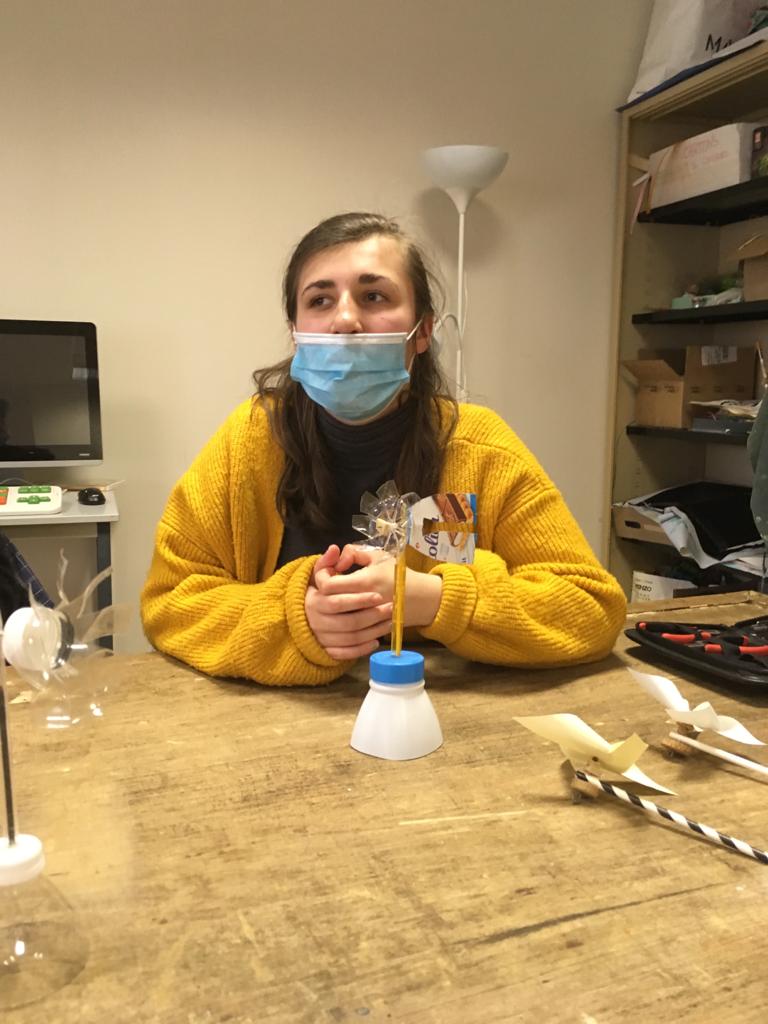In this image, an individual is seated in what appears to be their cozy home. They are surrounded by several pinwheels, each with a distinctive design; one features a striped pole while another is affixed to a plain white pole. Both pinwheels have white blades. Centrally positioned is a weather vane-style pinwheel with clear blades, accompanied by another similar pinwheel that seems diminutive, barely fitting on the tan table they are sitting at. The person is clasping their hands together, showcasing their long hair and a mask that only partially covers their face, leaving the nose exposed. They are draped in a gold cardigan that appears to be oversized. The backdrop includes a small table holding a computer and a colorful keyboard, implying a workspace. To their left, cluttered shelves brim with an assortment of knickknacks—potentially materials for making pinwheels, hinting at their passion for these whimsical objects. Additionally, a standing lamp is situated behind them, casting a warm light over the scene.